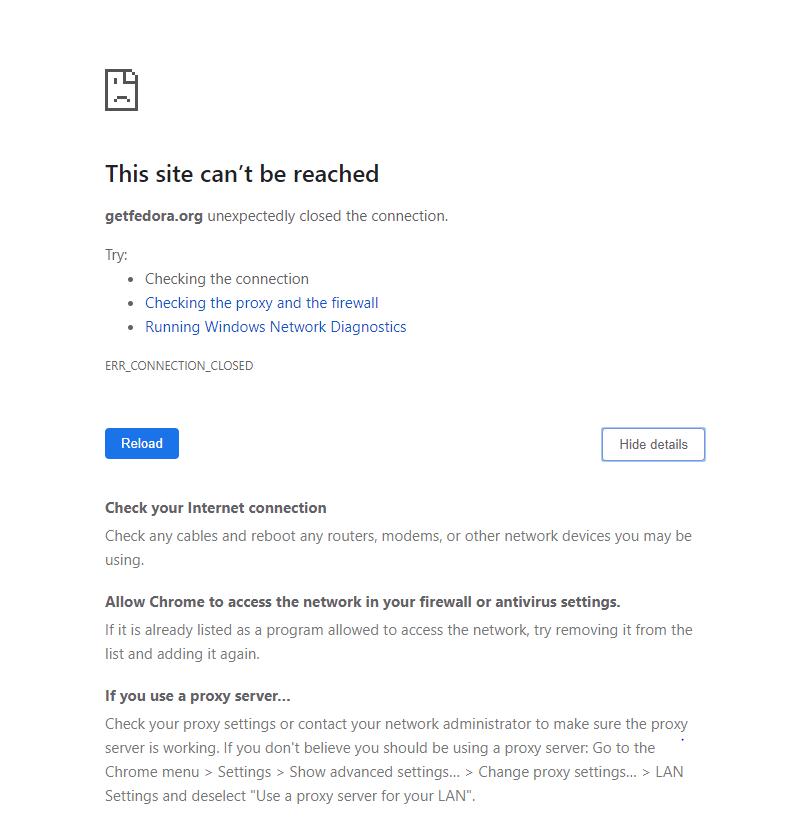A screenshot depicts a common web error message displayed in Google Chrome. At the top, a pixelated image of a frowning page icon indicates that the site could not be reached. Beneath this, the message "getfedora.org unexpectedly closed the connection" is prominently displayed. 

The error page provides potential troubleshooting steps: 
1. Checking the internet connection.
2. Examining the proxy and firewall settings.
3. Running Windows network diagnostics.

Below these suggestions, the error code "ERR_CONNECTION_CLOSED" is listed. 

Two buttons are visible at the bottom: "Hide details" and "Reload." The "Hide details" button appears to be inactive, revealing an expanded list of diagnostic steps. These include instructions to:
- Verify internet connection and cables.
- Restart routers, modems, and other network devices.
- Ensure Chrome can access the network through the firewall or antivirus settings.
- Remove and re-add Chrome to the list of allowed programs if necessary.
- Check proxy settings or consult a network administrator to validate the functioning of the proxy server.
- If unsure about using a proxy server, navigate to Chrome’s settings, access advanced settings, go to LAN settings under proxy settings, and deselect "Use a proxy server for your LAN."

This detailed error message aims to guide users through resolving connectivity issues effectively.